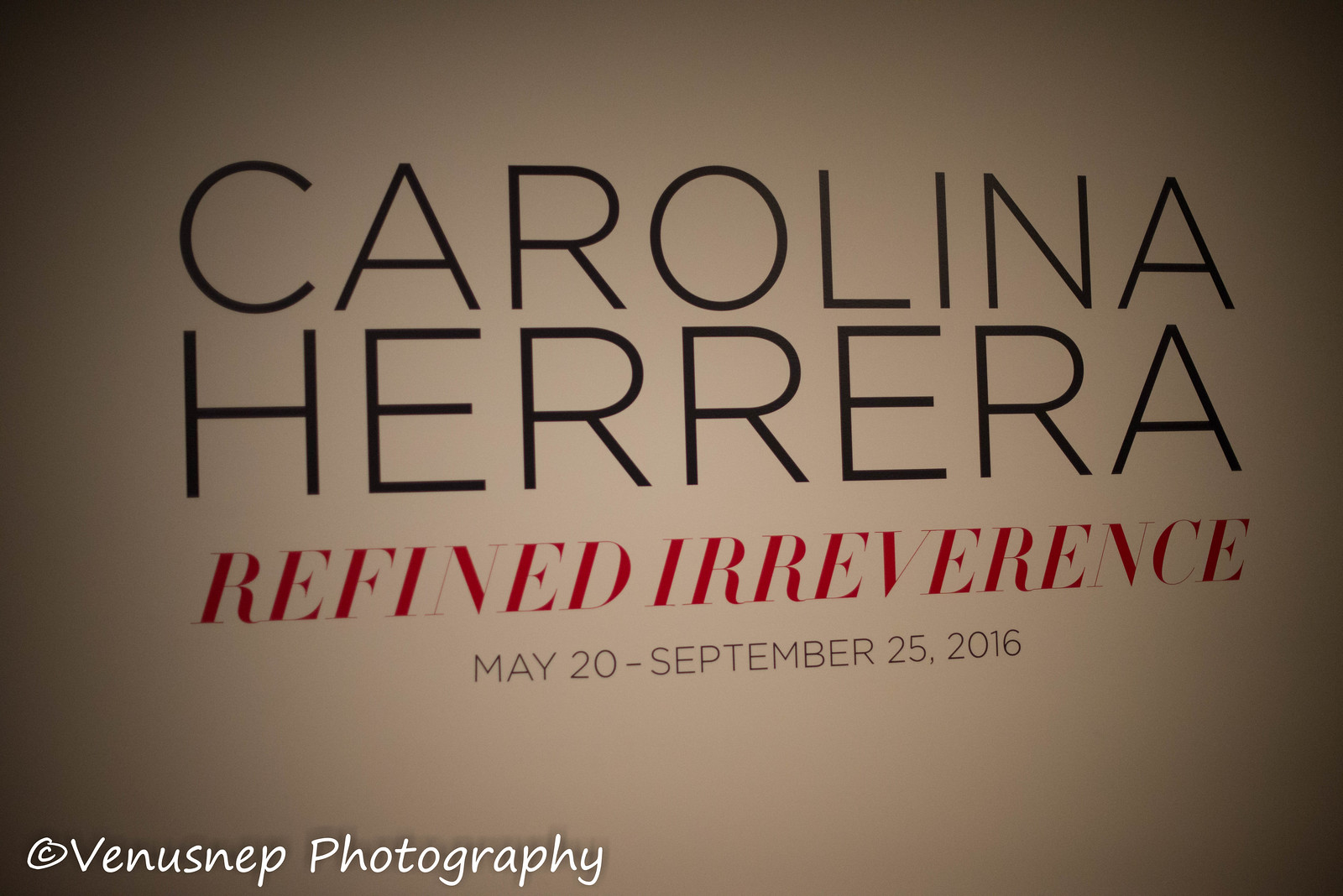This photograph displays a sign with a white background and dark edges, possibly printed on a wall or as part of an advertisement. Centered on the sign, in thin, black Arial font, are the words "CAROLINA HERRERA," all in capital letters. Below this, in bold, red serif font and also in capitals, it reads "REFINED IRREVERENCE." Further down, in a smaller black Arial font, the text shows the dates "May 20 - September 25, 2016." In the bottom left corner, there is a copyright notice stating, "Copyright Venus N.E.P. Photography." The overall setting around the sign appears to be dimly lit, enhancing the contrast and readability of the text.